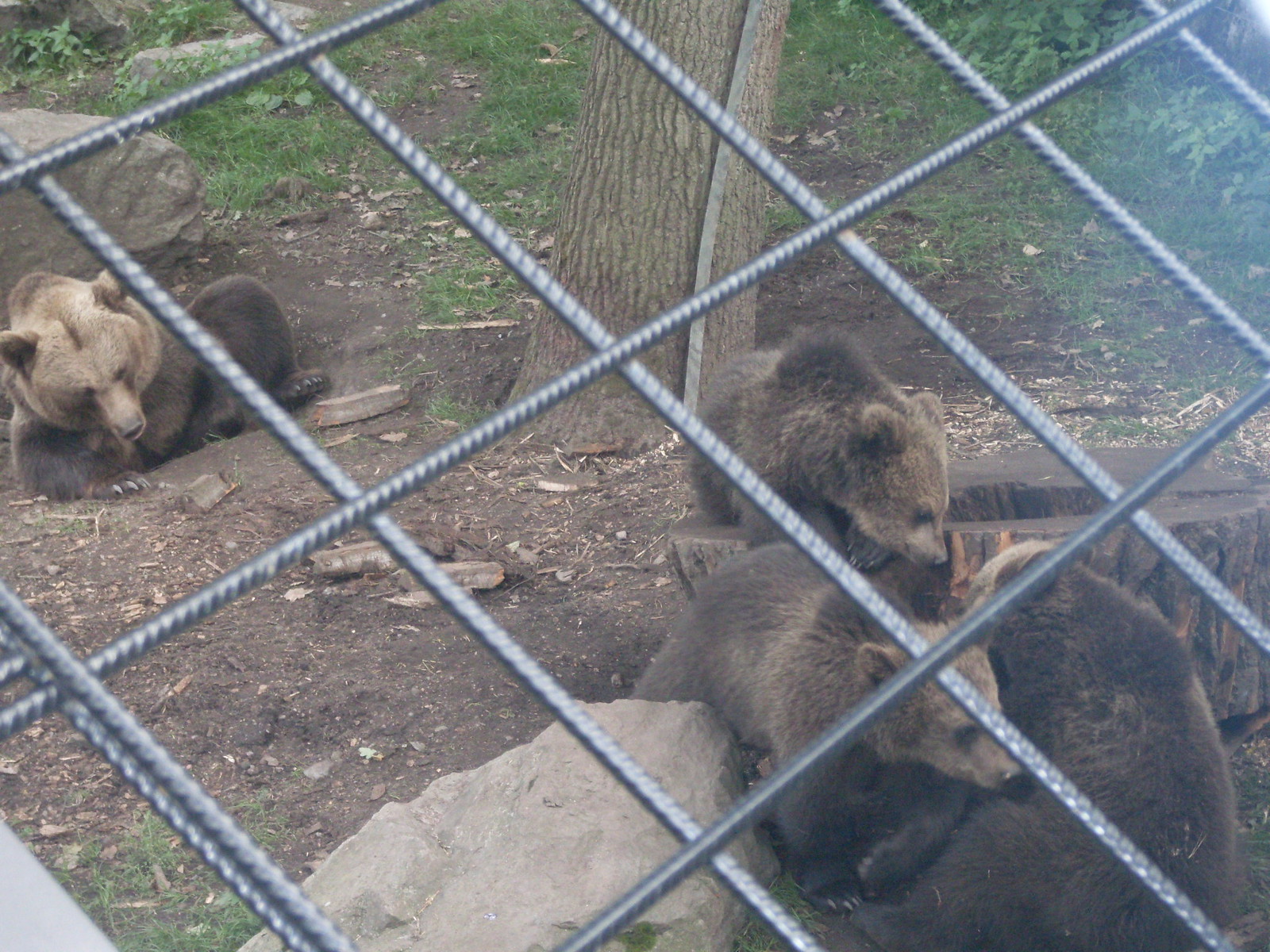The photo, taken through a cage-like structure with thick metal bars resembling rebar, captures a scene of four bears in captivity. In the upper left corner, a large brown bear with a lighter head and darker body is lying down, grooming itself, with its claws distinctively visible on both the left paw and back paw. This bear's snout is pointed towards the ground. In the bottom right corner, three bear cubs, perhaps only a few months old, snuggle together playfully. One of the cubs is partially inside a hollow tree trunk, which leans above the others, nestling its face into them. The cubs share the same color pattern as the larger bear, with light brown faces and dark brown bodies. The enclosure features a tree in the center, complete with hanging rope. The ground is mostly dirt, interspersed with small patches of grass and a prominent light-colored stone positioned in the bottom middle of the image, adjacent to where the cubs are located.